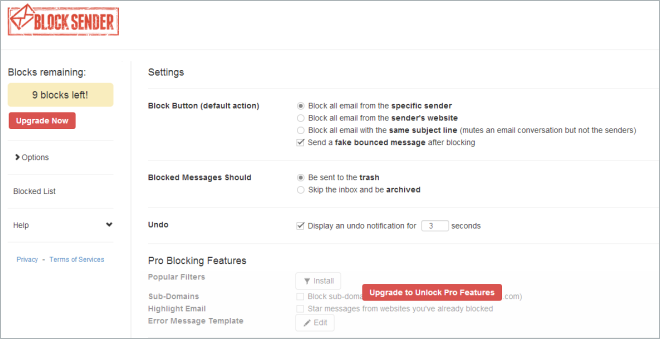A screenshot displays a user interface for blocking email senders. At the top, there is a bold red text stating "Block Sender," accompanied by an illustration of an envelope leaning against the letter "B." This section is enclosed in a red box. Below it are various menu options: "Blocked List," "Help," and "Privacy and Terms of Service," with the latter highlighted in blue and accompanied by a downward arrow.

To configure settings, the interface shows options such as "Block Button Default Action" with the choice to "Block all emails from this specific sender" checked. Another option, "Send a fake bounce message after blocking," is also checked. The configuration section continues with "Blocked messages should be sent to Trash," although part of the text is clipped. The option to "Undo and display an undo notification for three seconds" is selected.

The interface also includes a section for "Pro-Blocking Features" with popular filters. Additional options include a checkbox "Install" for enhanced features like subdomains, highlighting email, starring messages from already blocked websites, and an "Error Message Template" with an editable option. At the bottom, prominently within a red box, there is a notice stating, "Upgrade to unlock pro features."